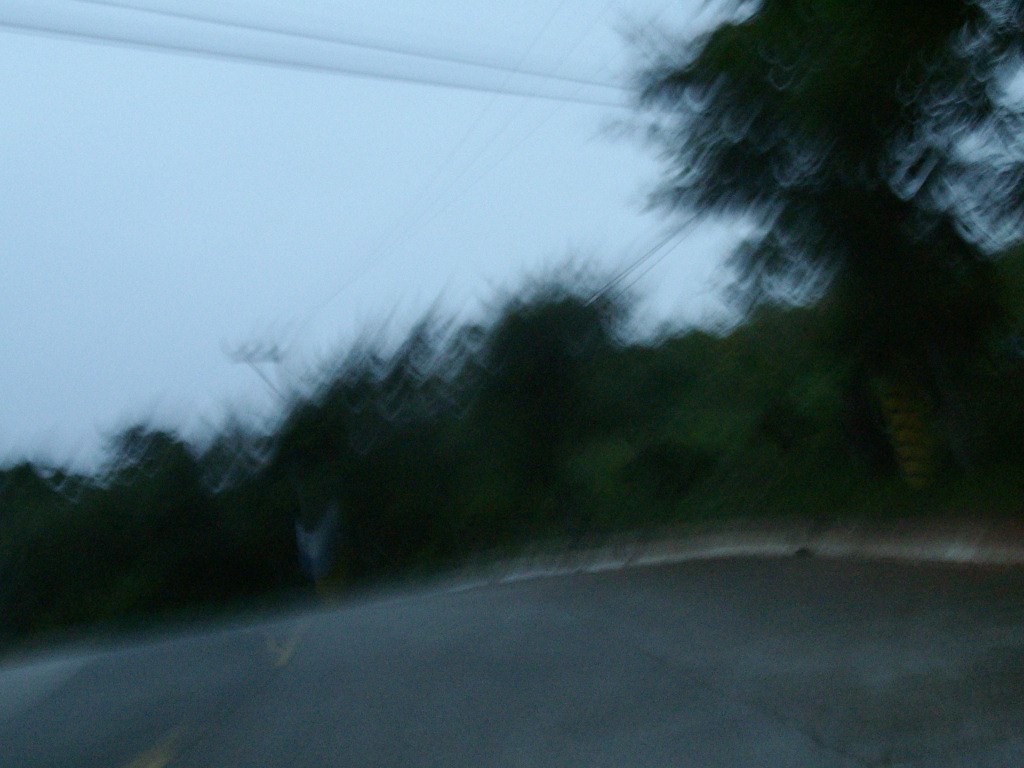The image captures a very blurry, black and white roadway scene that seems almost abstract due to its lack of clarity. The road, riddled with surface cracks, runs from the bottom right to the center left of the picture, bordered by a graystone curb. Above the curb, a towering tree contrasts sharply against the cloudy sky, which is marked by two sets of telephone wires stretching from the top left corner to the two o'clock position on the right. Across the center, a smaller tree line suggests a dense forest area ahead, making it seem like the road leads directly into a multitude of trees. The sky appears dark and overcast, possibly influenced by the windy or rainy conditions suggested by the blur effect. Amidst the shadows of the shrubberies, there is a faint outline of a small animal nearing the curb, adding an element of life to this otherwise desolate and blurred twilight scene.